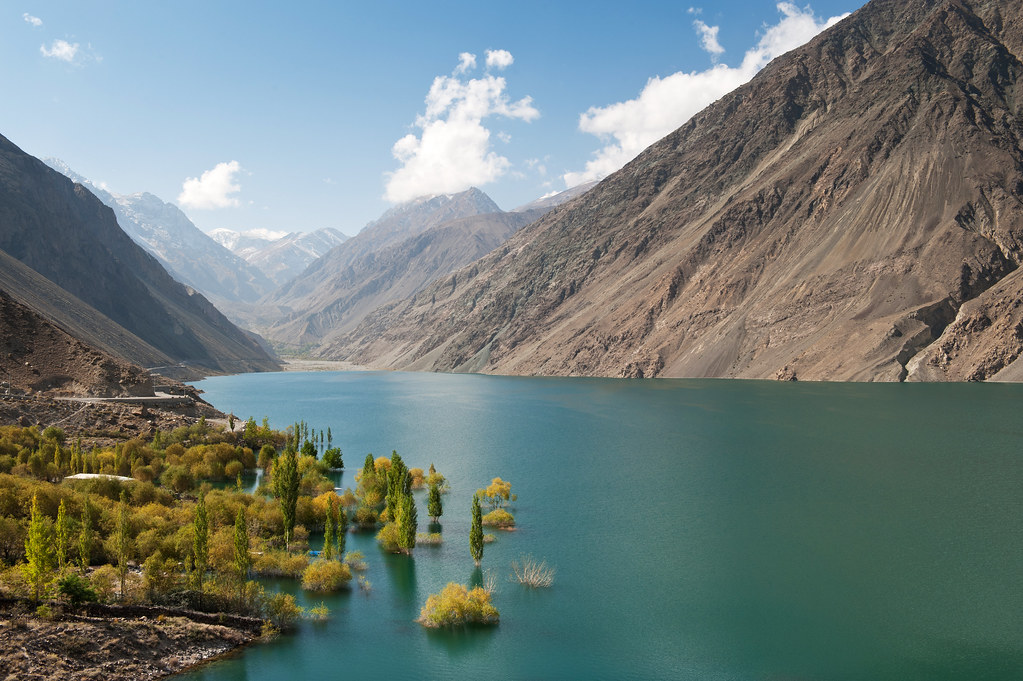Perched high above, this detailed aerial view captures a breathtaking mountain landscape surrounding a serene, blue-green lake. To one side of the lake, rugged grayish-brown mountains stand tall, while the opposite side teems with dense greenery, a mix of trees and various tall bushes. A well is visible among the foliage. The lake lies almost still, its tranquil surface mirroring the pristine blue skies dotted with a few scattered clouds. At the far end of the lake, a small valley slices through the mountains, hinting at an extended passage through this vast, majestic range. The vegetation along the water's edge exhibits a diverse palette, transitioning from vibrant green to shades of yellowish-green, although the area appears devoid of visible wildlife. This expansive view, taken from an elevation of around 300 to 400 feet, offers a partial glimpse of the lake's grandeur, leaving much more of its beauty to be imagined beyond the frame.